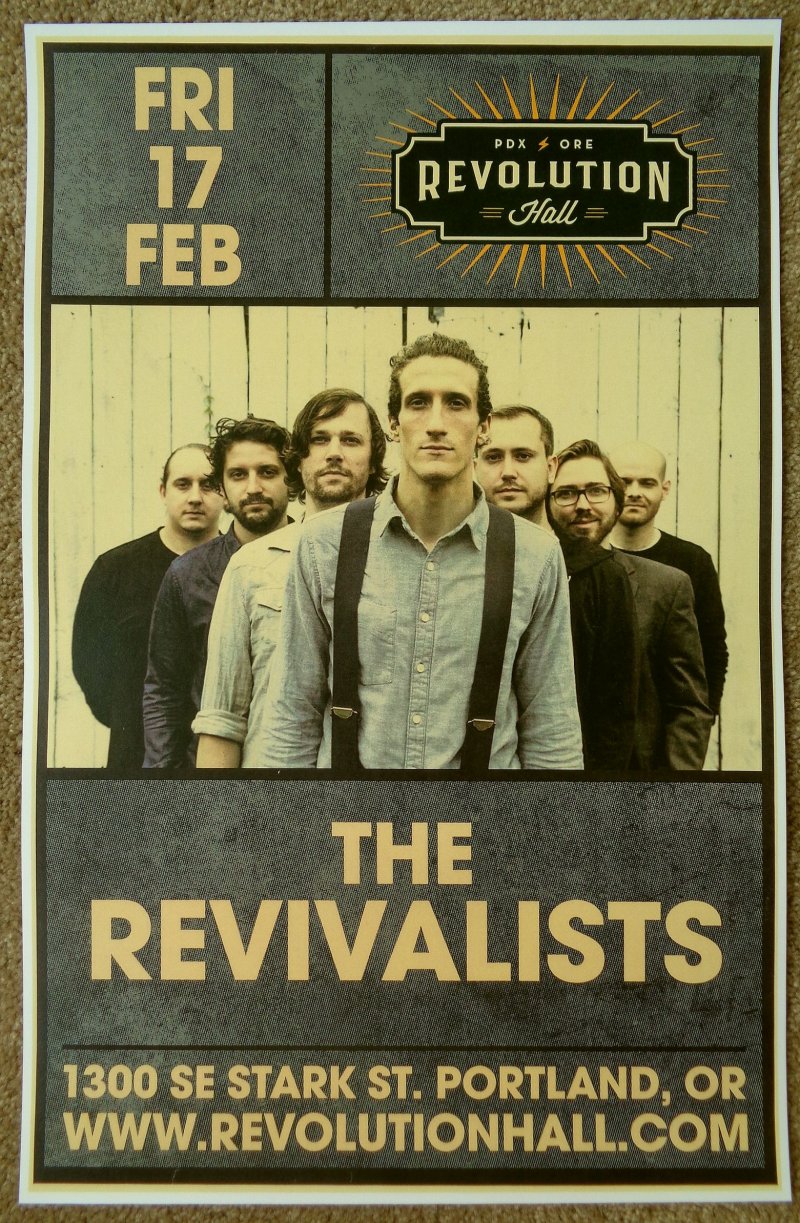This vivid poster advertises a performance by the band The Revivalists at Revolution Hall, located at 1300 SE Stark St, Portland, OR. The show is scheduled for Friday, February 17th. The top left portion features a dark blue background with pale yellow text that reads "Fri 17 Feb," while the top right displays the Revolution Hall logo, also set against a dark blue backdrop with orange spikes emanating outward and pale yellow text. At the bottom of the poster, the band's name and the venue's address www.revolutionhall.com are listed in a matching light tan color.

Dominating the center is a sepia-toned photograph of the seven-member band, all light-skinned males with brown hair. They stand in a staggered formation against what looks like a white barn. The lead singer is front and center, wearing a blue shirt and suspenders, surrounded by his bandmates clad in dark-colored sweaters, shirts, or jackets in hues of navy, blue, brown, or black. Among them, three sport beards, one has glasses, and another has just a mustache. These details create an evocative image of the band’s classic western attire and rustic aesthetic, making the poster both informative and visually striking.